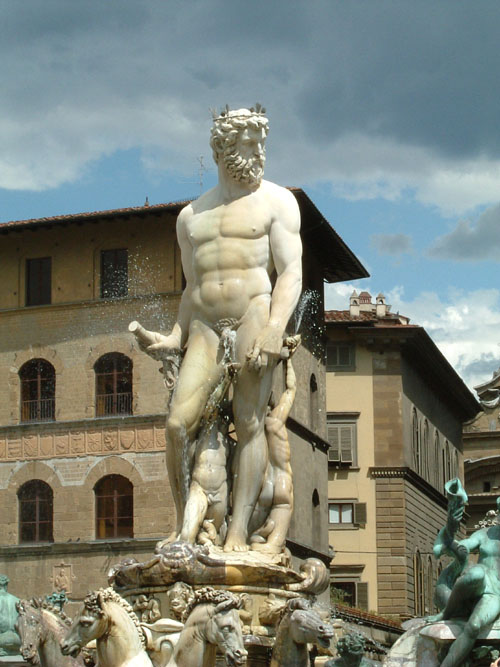The image depicts an imposing, intricately detailed marble statue set in an outdoor fountain, viewed from a low angle. The central figure is a nude, muscular bearded man adorned with a crown or wreath, holding a cylindrical object. He stands with water cascading around him, surrounded at his legs by entwined cherubic children, possibly toddlers. Below him, four horse heads emerge, adding to the fountain's elaborate design. The statues, predominantly white marble, include a few green verdigris-covered figures, indicating some of the material may be copper. Positioned in an urban area, the fountain is framed by several old, possibly European sandstone-colored buildings with arched windows and intricate carvings, reminiscent of ancient Roman architecture. The sky is partly cloudy, with patches of blue peeking through, illuminating the scene with a gentle, sunlit ambiance.